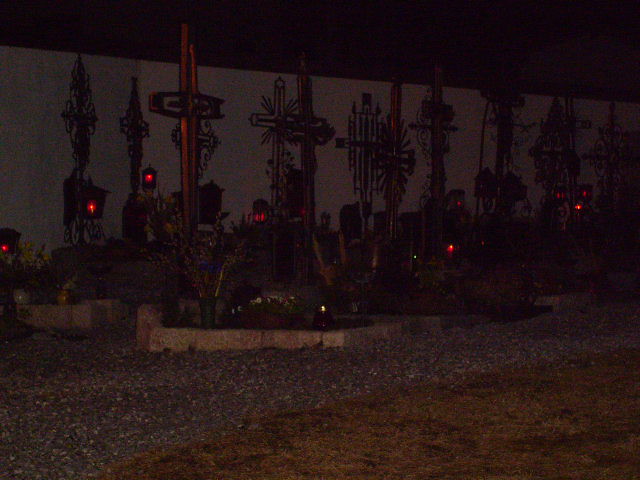This nighttime photo depicts a yard or grounds area, possibly a memorial or foreign graveyard. The scene features numerous cross-shaped and elegantly designed metal figures standing tall amidst small, circular gardens bordered by white concrete blocks. Each garden contains green and yellow plants, with some having lanterns emitting red light. The ground alternates between brown grass or dirt and gray stone gravel. In the background, a tall white concrete wall is visible, contrasting with the dark sky above. Rows of large crosses, crafted from both wood and metal, stand solemnly in the dimly lit garden, creating an atmosphere of somber elegance.